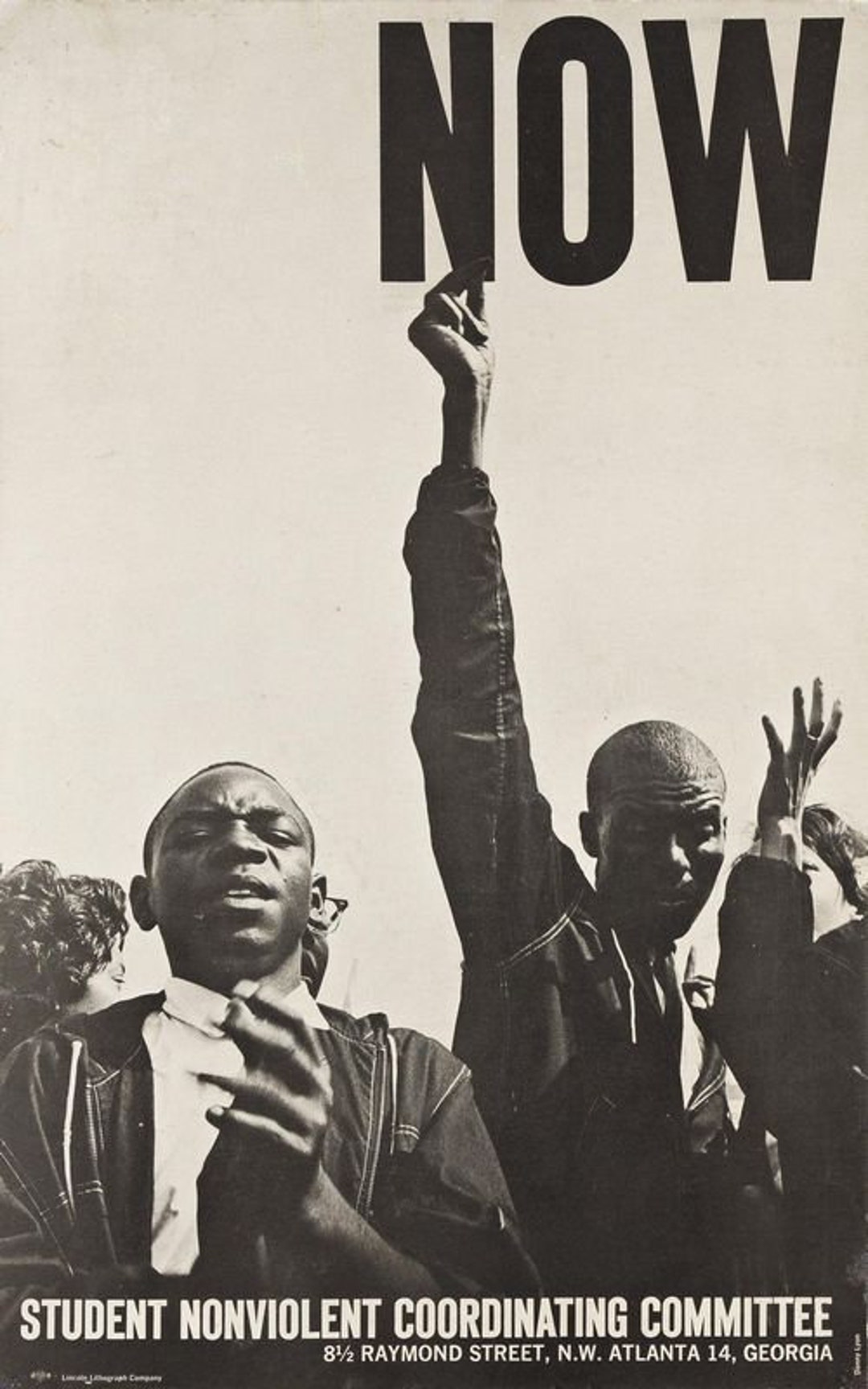The image appears to be an old black-and-white poster for a protest organized by the Student Nonviolent Coordinating Committee, located at 8 1⁄2 Raymond Street, Northwest Atlanta 14, Georgia. The focal point of the image is a small group of African American individuals, with two men prominently in the foreground. The man on the right is standing with his arm raised high, his fingers snapping just below the large black letters spelling "NOW" in the upper right corner. The man on the left is clapping with a serious expression on his face. Both men are dressed in jackets, dress shirts, and ties. Behind them, partially visible, are more individuals including a woman with her hand raised. The overall tone of the image is sepia, adding to its vintage feel.